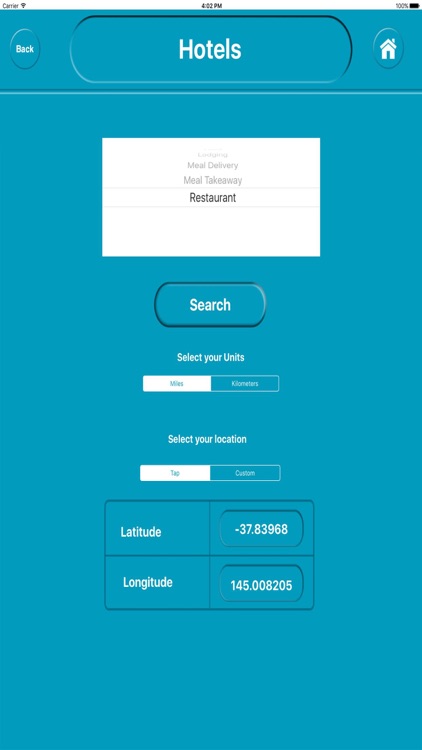The screenshot appears to be from a mobile application, displaying the interface in clear and vibrant quality, albeit with some elements rendered in small font. At the top of the image, there is a status bar featuring a Wi-Fi icon, a slightly indistinct time, and a battery percentage indicated as 100%. Below the status bar, there is a section in a shade slightly darker than Tiffany blue, containing several functional elements in white font. 

Towards the left, there is a blue button emblazoned with the word "Back." Centrally, there is a broader button with the word “Hotels” and a small icon of a house within a blue circle. 

Further down, a white box appears to outline meal options, and within this section, the word "Restaurant" is prominently shown in black text. Beneath this, a blue and white search bar reads "Select your units," accompanied by white and blue selection boxes. Similarly, below this, another prompt reads "Select your location," alongside corresponding selection boxes. The interface also displays specific geographical coordinates: 37.83968 for latitude and 145.008205 for longitude. 

Though the image quality is clear, the small size of certain text elements makes it difficult to read all details with utmost clarity.